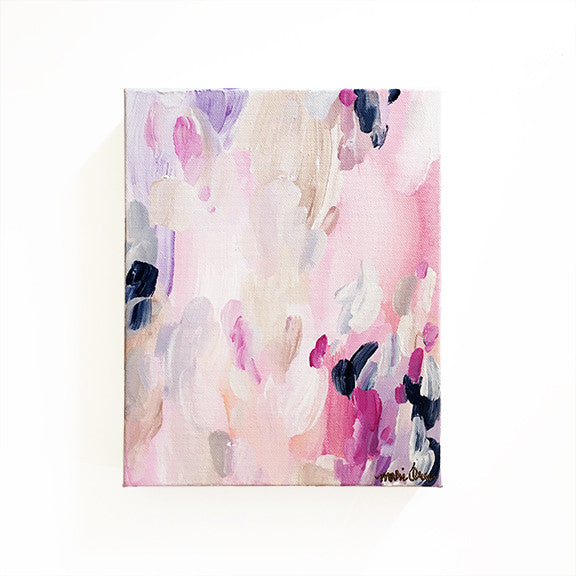This is an image of a small, square-shaped painting, approximately 4 inches high and 4 inches wide, displayed on a white wall that casts a subtle yellow shadow. The painting, on a canvas around 2 inches wide by 3 inches high, features a variety of thick, overlapping brushstrokes in predominantly pastel colors. The palette includes shades of pink, purple, cream, tan, and sparse touches of black. Brushstrokes vary in direction, creating an impressionistic scene that, with imagination, could be interpreted as an abstract collection of flowers or petals. There is a notable concentration of colors in the lower right corner, where the artist has signed their name in cursive—though the name is partially illegible, appearing to be either "Modi" or "Moby." Patches of black paint are sporadically placed in the center left, upper right, and lower right corners, enhancing the contrast against softer hues. The blend of colors and the dynamic brushstrokes give the piece an expressive and versatile aesthetic suitable for various decorative settings.